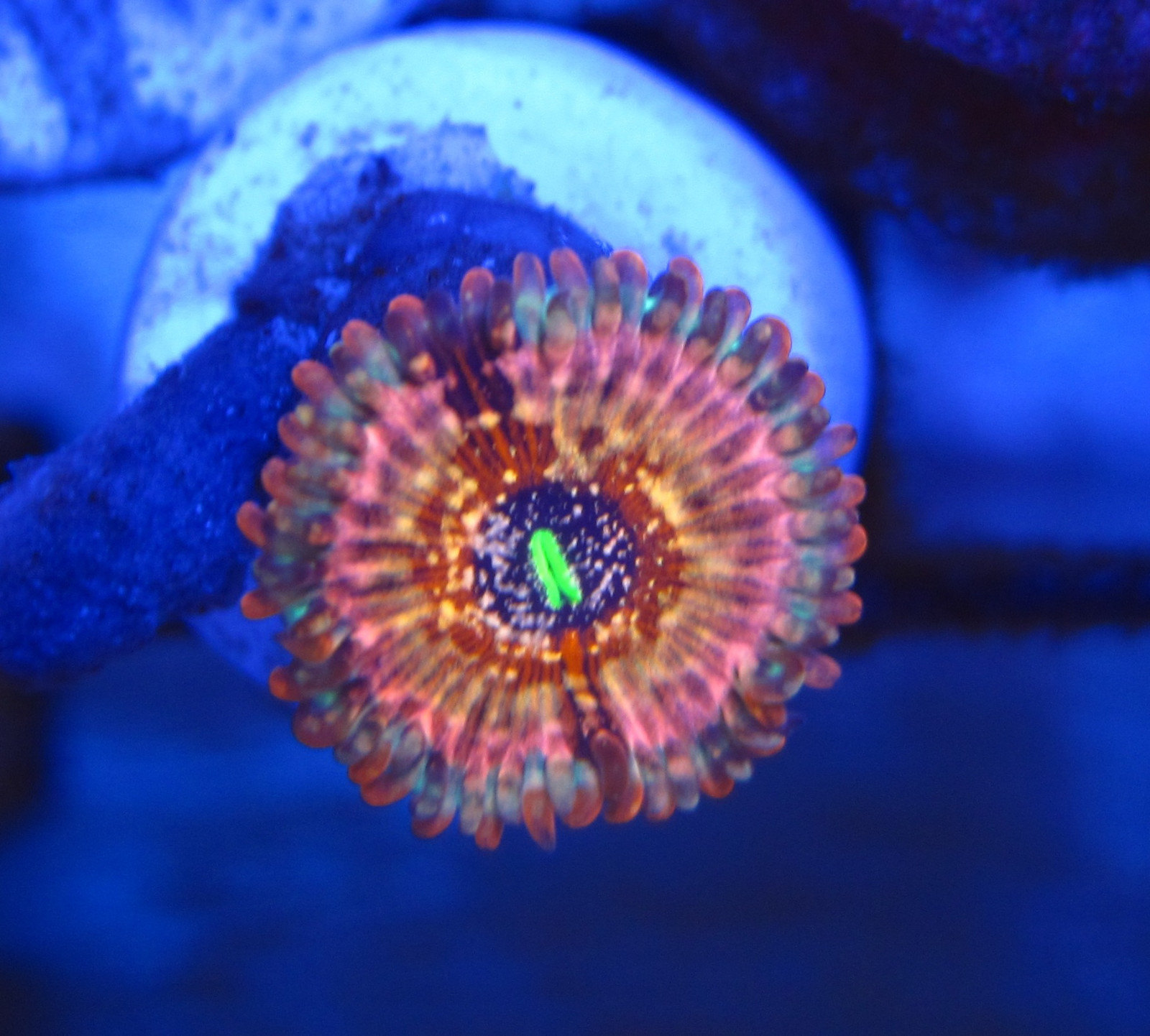This image depicts an underwater scene featuring a bioluminescent organism that resembles both a flower and a sea creature. Central to the image is a vibrant, luminescent structure with a neon green core surrounded by red and yellow specks that transition into pink, orange, and purple hues. These colors are segmented by a dark black band and extend outward into what appear to be delicate, cilia-like structures. The outer fringes of these "petals" or tendrils are tinged with blue and purple shades, giving the appearance of a living, pulsating sea anemone. The backdrop of the image is an ethereal expanse of blues and purples, suggesting an underwater setting. Additionally, there is a light blue, stem-like feature emerging from beneath the organism, contrasting against the darker, blurry, and unfocused background, which enhances the surreal and almost alien beauty of the scene.